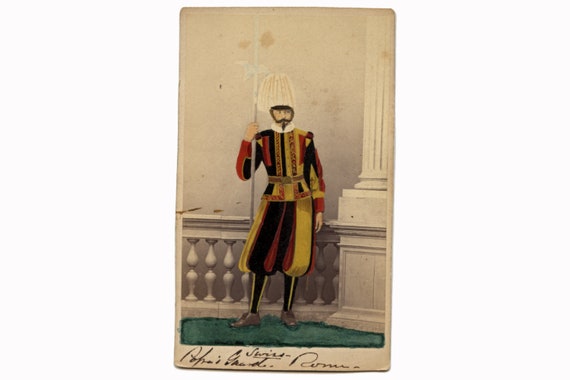This is a detailed, full-color vertical painting without a distinctive border, set indoors against a backdrop of grayish off-white marble walls, columns, and a balustrade. The artwork depicts a member of the Swiss Guard, historically tasked with defending the Pope. The guard is a bearded, mustachioed white man in his 30s, wearing the iconic, elaborate uniform of the Swiss Guard. This includes yellow, red, and black striped puffy knickers and a matching long-sleeved military-style tunic, secured by a brown belt. His black and white striped socks are paired with brown lace-up boots. He is crowned with a tapered white hat and holds a spear in his right hand. The image features cursive text, likely identifying the subject as "Swiss Guard" and possibly "Pontifical Roman" or a similar phrase. Despite a visible artist's name at the bottom, it remains unreadable. The spear he holds is adorned with a blade resembling an axe, completing his ceremonial, yet formidable, appearance.